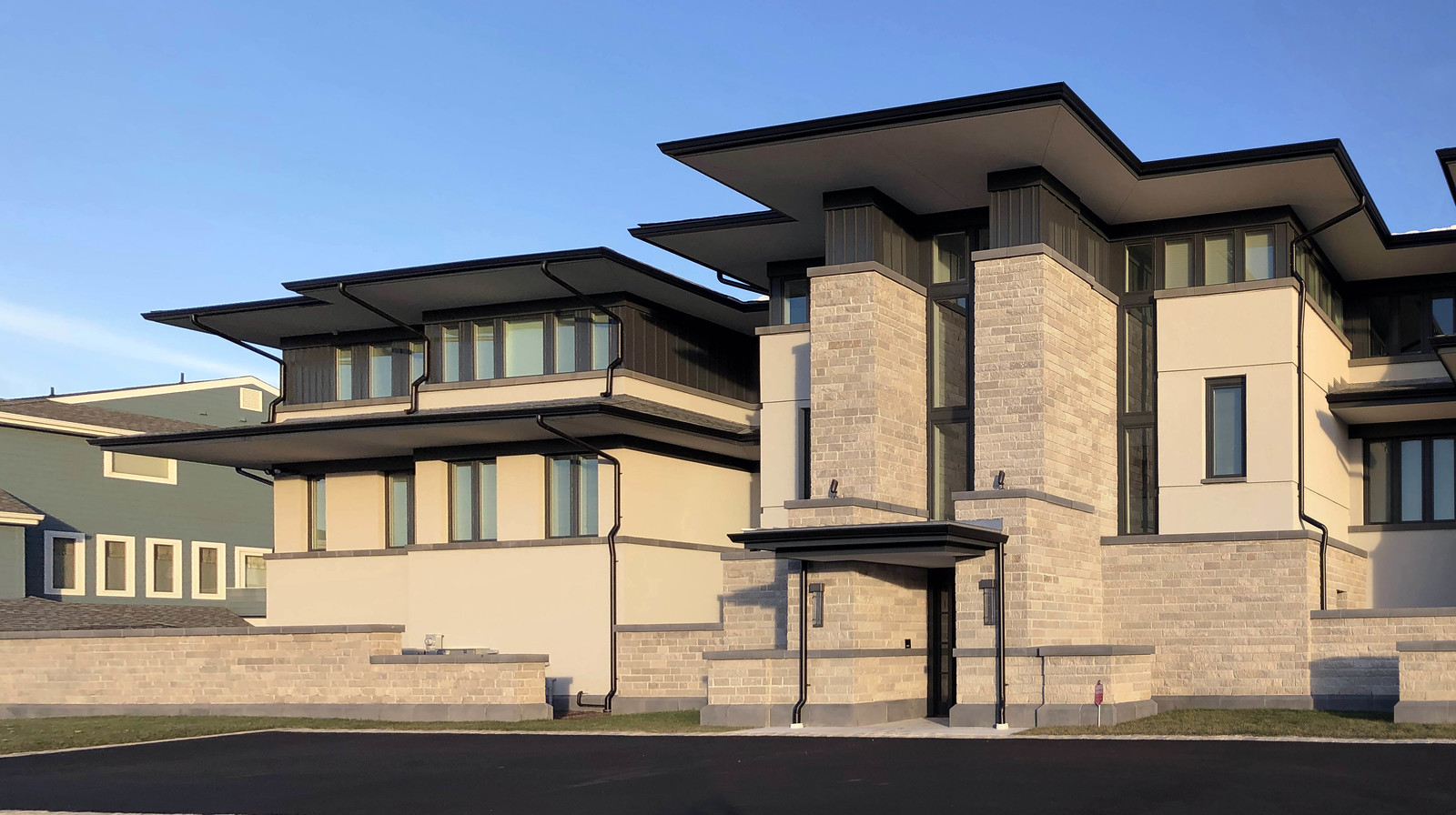This daytime outdoor image features a large multi-story building as the main focus, set against a clear blue sky with only a faint, wispy cloud or contrail near the center left. The building boasts a flat roof and a symmetrical design accentuated by numerous, closely-set rectangular windows, surrounded by a very dark brown trim. The facade artfully combines earthy tones, with prominent brick pillars and sections of vanilla-colored siding. To the left, brick walls add to the cohesive, muted color palette. In the far left and center of the image, you can see another separate building, characterized by a bluish-gray hue and white window frames. Despite an overall simple appearance, the image hints at a digitally-rendered perfection, enhanced by the surrounding patches of greenery.